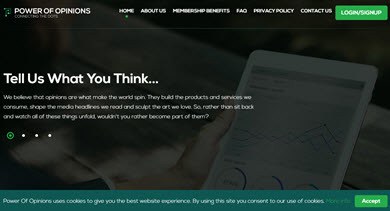The image shows a detailed screenshot of a webpage, seemingly minimized to a very tiny size. In the upper right corner, the text "Power of Opinions" is barely visible. At the top of the page, there's a menu bar with navigation links, including Home, About Us, Membership Benefits, FAQ, Privacy Policy, Contact Us, and Login/Sign Up. Under this menu, a graphic depicts a person holding up a tablet displaying a graph. Above the graphic, a heading reads "Tell Us What You Think." Below this section, there is a paragraph of text that is too small to be read in the image. The webpage appears to be part of a slideshow, with this being the first of four slides. At the bottom, there is a green bar containing an Accept Cookies banner. The image itself does not show any taskbar or search bar, focusing solely on the webpage. The layout is in a widescreen format, slightly wider than the standard 16:9 ratio.